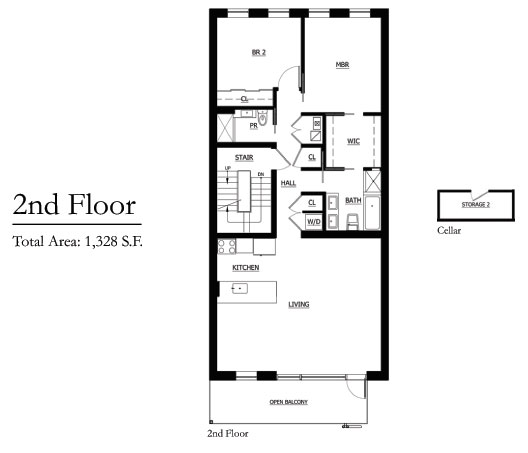This detailed floor plan illustration showcases the second floor of a home and its accompanying cellar. On the left side of the image, the label "Second Floor" is clearly displayed, with an additional note underneath indicating the total area as 1,328 square feet. To the extreme right, a small black box marked "Storage Tube," with "Cellar" noted beneath, signifies the cellar area.

The second floor plan is encompassed within a black box that meticulously details the layout of various rooms. Visible rooms include a living room, a kitchen, a bathroom, a laundry room, and two bedrooms. The plan also indicates a second bathroom and a designated washroom. The location of the stairs leading down to the first floor is clearly marked.

Additionally, at the bottom of this floor plan, an "Open Balcony" is noted, indicating that there is an accessible outdoor space at the end of the living room, providing a place to step outside and enjoy the view from the second floor. This comprehensive plan gives a clear and detailed overview of the home's second floor and cellar layout.